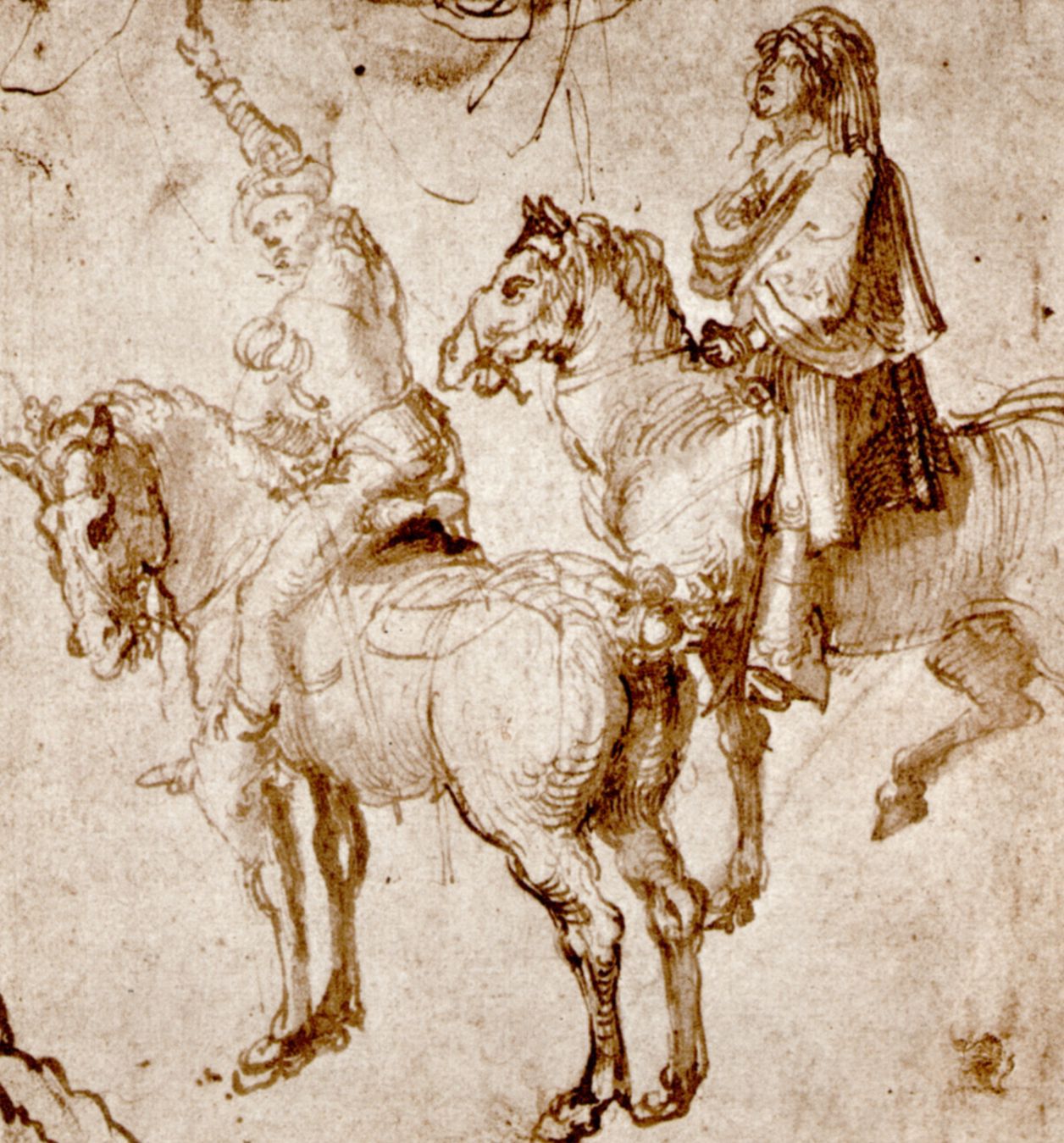This image is a hand-sketched drawing by Albrecht Dürer, titled "Studies by Two Writers," created in 1499. Rendered in orangish-brown sepia tones on a beige and light brown background, the square-format drawing showcases two horses and their riders. The central horse, seen from its left side, is predominantly beige with dark brown outlines accentuating its back, legs, and face. Mounted on this horse is a man in a soldier's uniform, featuring puffy sleeves and armor down his back. He is turning to look over his left shoulder, with his right arm upstretched and his left arm bent in front of his waist. His left leg drapes over the horse’s side. 

Behind the central horse is another horse facing left, also with dark brown outlines along its mane, head, and limbs. The rider of this second horse wears a caped garment and a veil, with dark brown detailing on their backside. They are positioned more upright, with their head tilted back and their right arm held at their chest. The entire scene is set against a vague backdrop marked by dark brown, scribble-like lines that suggest tree branches above. The artwork is characteristic of Renaissance Gothic art and captures an ambiance that hints at past centuries, specifically the 18th or 19th century.